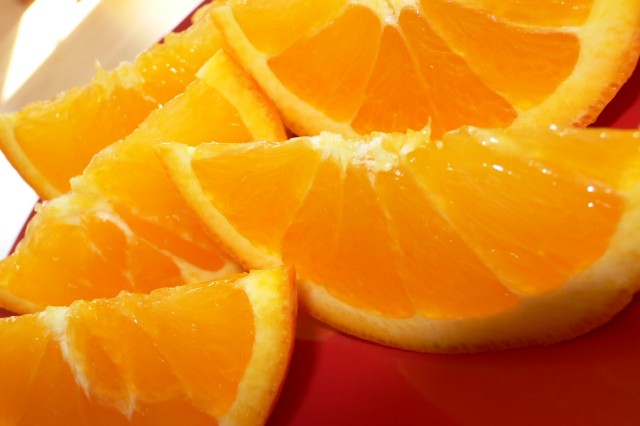The close-up, high-quality photograph captures a cluster of vibrant, juicy orange slices resting on a bright red surface, almost completely obscuring what is likely a plate. The image is taken at a slightly crooked angle, adding a dynamic feel, with the orange segments arranged tightly together. The segments are half-circles, with their straight edges pointing upwards. Some slices show the white pith and thin peel, and there are highlighted areas on the pith along with subtle shadows suggesting the source of light. The bright orange flesh contrasts vividly with the red background, accentuated by the overall excellent lighting. In the upper left corner, there is a hint of a light-colored surface, possibly a table, contributing to the well-lit setting. This detailed composition makes the orange slices appear particularly appetizing and inviting.